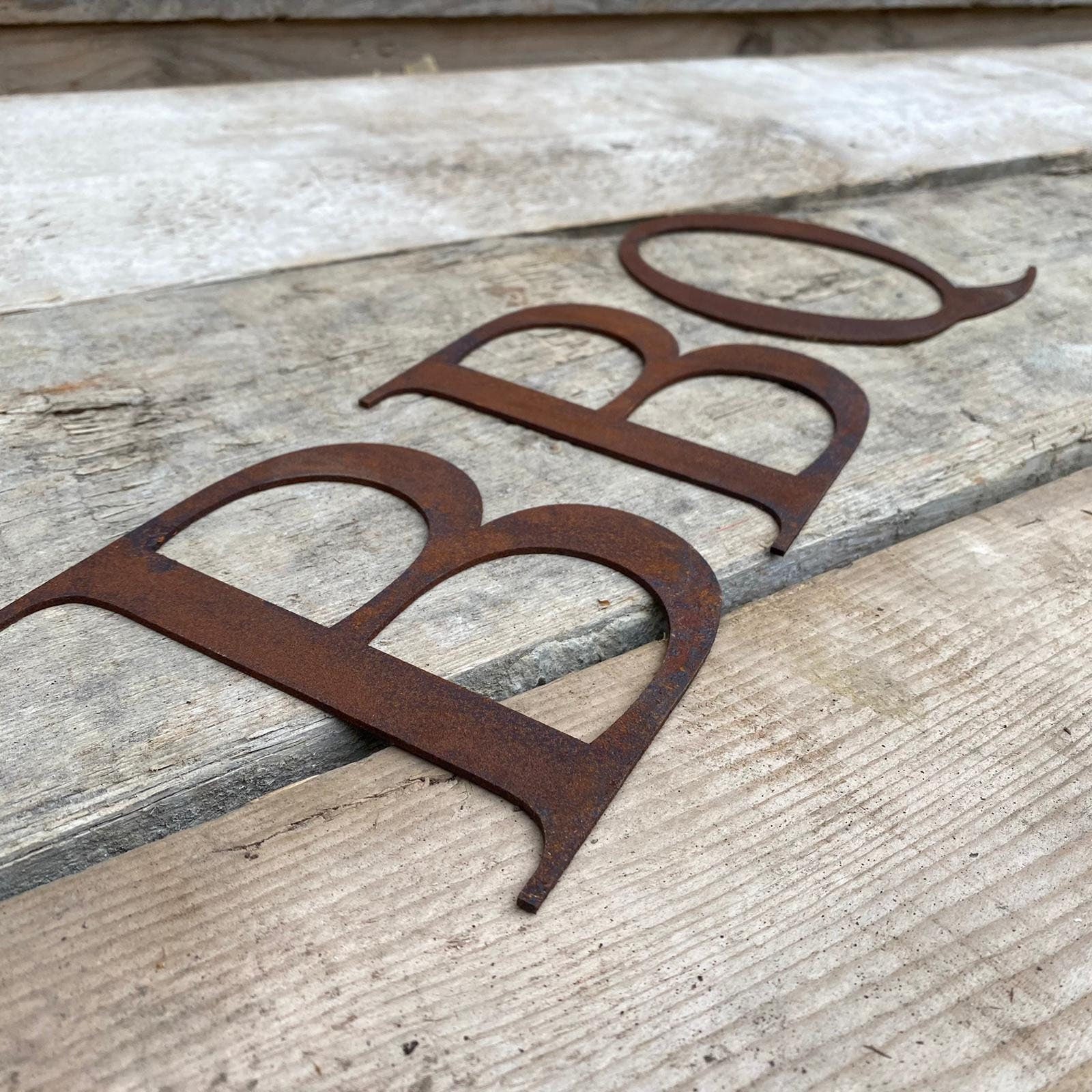In this image, there is a close-up, angled side view of three rusted metal letters spelling out "BBQ," arranged on an aged wooden deck. The image, likely taken outdoors, captures the letters from a slightly above and left perspective. Each letter, approximately three inches tall and two inches wide, is crafted from thin sheets of steel showing a reddish-orange rust with some black metal visible beneath. The deck, composed of three two-by-six planks, has a weathered grayish tone with visible grain, cracks, and splinters, adding to the rustic atmosphere of the setting.